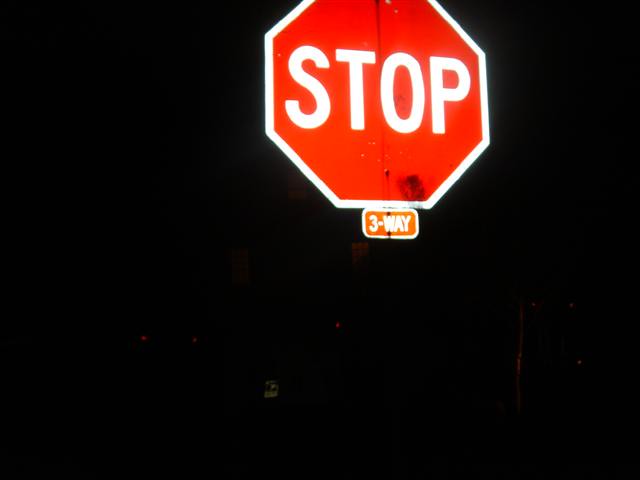This photograph, taken at nighttime, depicts a vibrant, illuminated stop sign prominently centered against an almost pitch-black background. The stop sign is an octagonal shape, characteristic of American traffic signage, featuring a bold red background with "STOP" written in large, white capital letters. Surrounding the red octagon is a distinctive white border, and directly beneath the main sign, a smaller sign with a similar red background and white text indicates "THREE-WAY," identifying it as a three-way stop. The sign is strikingly illuminated by bright headlights, causing its reflective elements to stand out sharply, making it appear as if it's floating in the darkness. In the background, several faint red lights are visible, likely belonging to distant vehicles or possibly the outline of a bus. On the right side of the image, a vague box-like shape with a white sticker is faintly noticeable, hinting at a post office box. The scene is dominated by the contrast between the illuminated stop sign and the enveloping darkness.